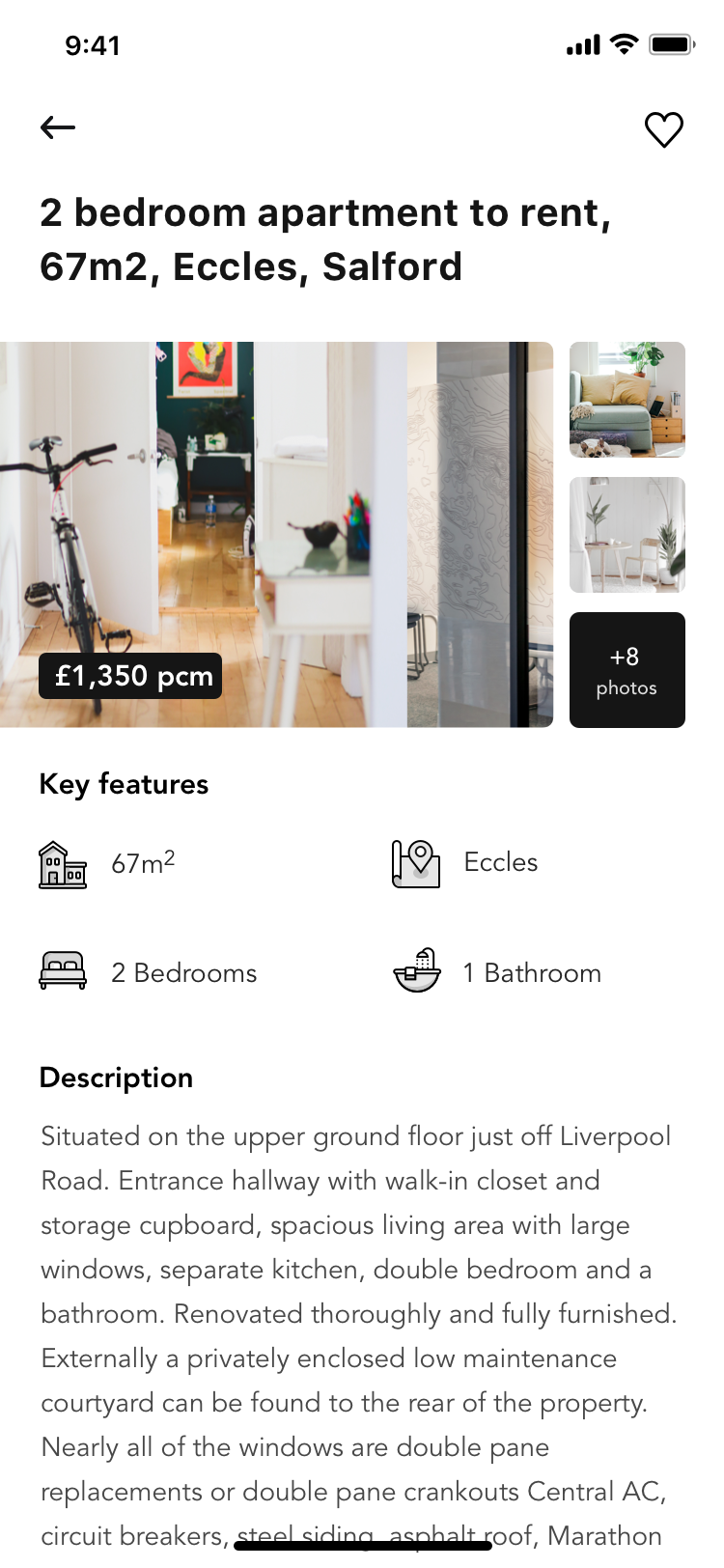**Advertisement Image Description: Spacious Two-Bedroom Apartment for Rent**

The image showcases an advertisement for a rental property prominently displayed at the top of the page. The headline reads: "Two-Bedroom Apartment to Rent, 67m², Eccles, Salford." The structure of the text uses the numeral "2" for the bedroom count.

The advertisement appears to be a screenshot from a mobile device, indicated by the back button in the top left corner and a heart icon in the upper right. Above these icons, there is a timestamp showing "9:41," along with the device's Wi-Fi and battery status.

Below the headline, there is a main image of an apartment interior, which includes a partial view of a hallway with a bike and a bedroom in the background. The rent is listed as "£1,350 PCM" (per calendar month). To the right of this main image, there are two smaller images and a label indicating "plus 8 photos" against a black background in the bottom-right corner.

Further details are provided below the images under the heading "Key Features." The building is noted to be 67 square meters and located in Eccles. It features two bedrooms and one bathroom.

The description elaborates, "Situated on an upper ground floor just off the road, the apartment includes an entrance hallway with a walk-in closet and storage cupboard, a spacious living area with large windows, a separate kitchen, a double bedroom, and a bathroom. The property has been thoroughly renovated and comes fully furnished. Externally, there is a privately enclosed low-maintenance courtyard at the rear of the property."

Additional amenities include nearly all windows being double-pane crank outs, central air conditioning, circuit breakers, steel siding, and an asphalt roof.

The advertisement concludes with this information, providing a detailed and comprehensive overview of the rental property.